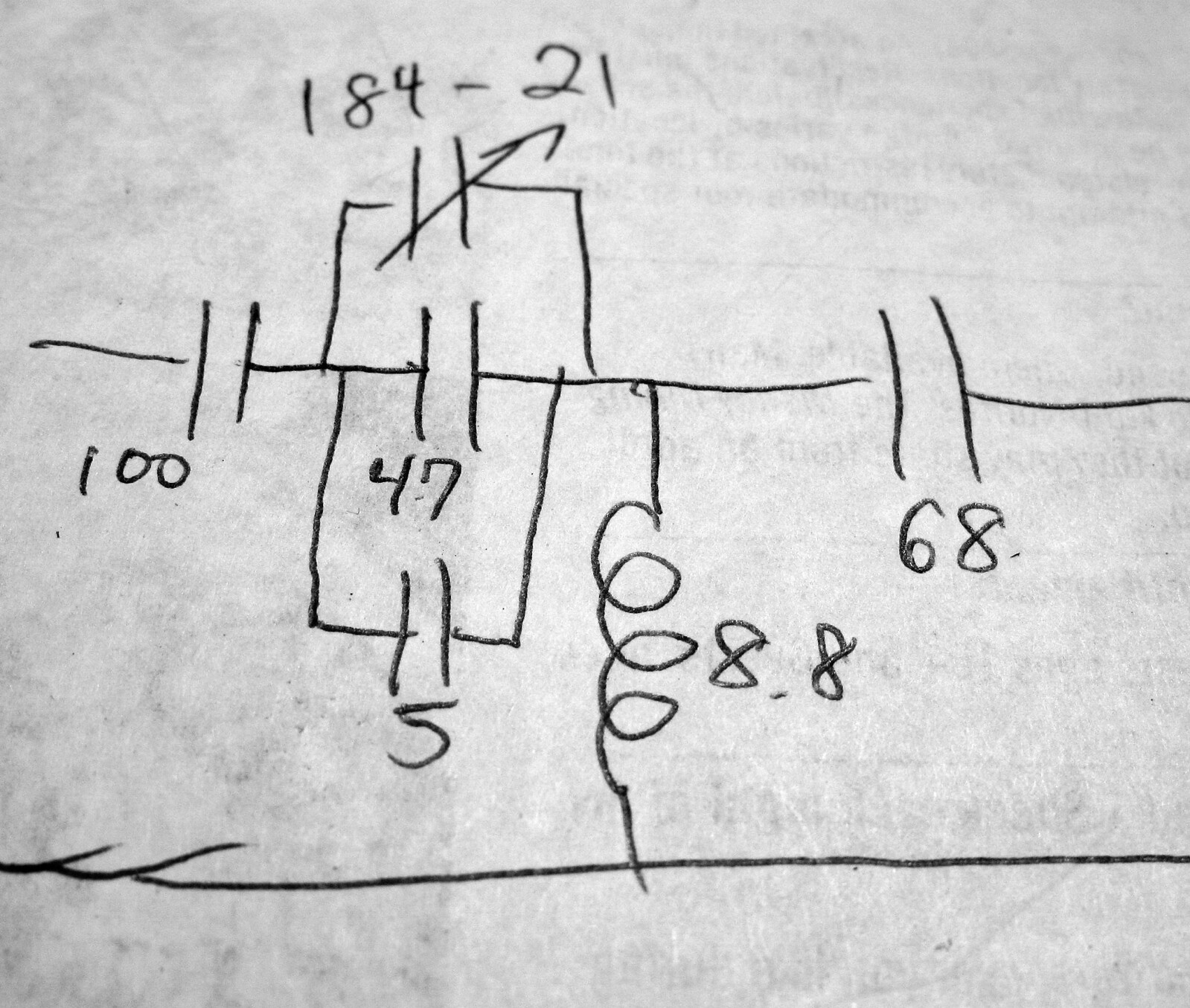On a gray and white mottled background, likely bearing remnants of ink from a previous print, an intricate diagram unfolds with precision. At the top of the diagram, the numbers "184-21" are prominently displayed. Beneath this identifier, the diagram appears to be part of an electrical schematic.

Black ink lines traverse the document both horizontally and vertically, mapping out connections and pathways. At the top center of the diagram, a square is segmented by vertical lines, leading upwards to an arrow that points directly to the number "21."

Adjacent to this top square and reaching towards the bottom, a series of black lines intermingle. To the left, the number "100" is marked, while just right of it, a spiraling line descends to the notation "8.8." Just above this spiral, another set of vertical lines is annotated with "68."

Prominently, another square at the bottom center houses the number "47," beneath which is the number "5." Below these elements runs a horizontal line stretching from left to right; it features two small upward swoops on its left side. The aforementioned spiral intersects this horizontal line, piercing through its center.

Together, these elements form a complex and detailed schematic, rich in numerical and graphic detail, against a textured backdrop that hints at its unique and perhaps reused origins.